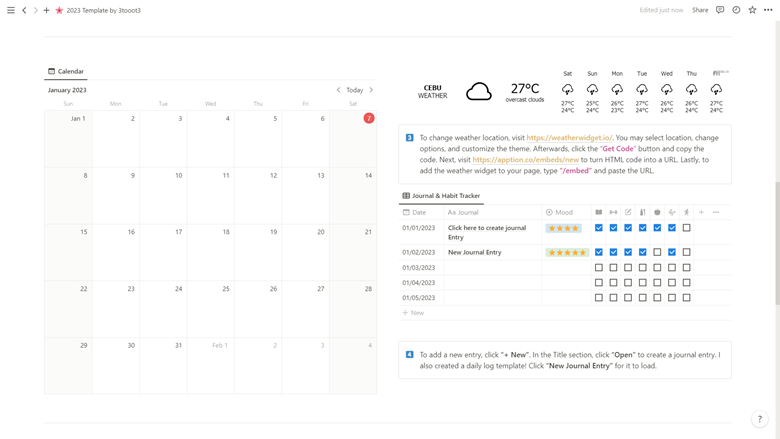The image depicts a calendar template for January 2023, featuring a light gray border. On the right margin is a thin gray scrollbar. At the top, above the calendar, a navigational toolbar includes three horizontal lines, forward and backward buttons, a plus sign, a star icon, and the gray text "2023 template by J...", with the full name partially obscured. To the far right, it says "edited just now" in light gray text, alongside icons for favoriting and a three-dot menu for more options.

The calendar itself is positioned on the left and shows January 2023, starting with Sunday, January 1st. Notably, Saturday, January 7th is highlighted with a red circle around the date. Weekdays are presented in white boxes, while weekends (Saturdays and Sundays) are shaded in light gray.

The right side of the image features a weather report for Cebu at the top. It displays a cloud icon with the text "27°C" and "overcast clouds" below it. The daily weather forecast for the upcoming week is also included, indicating cloud and rain icons for each day from Saturday through Friday.

Below the weather report is a section within a white box bordered in gray, containing information on how to change your weather location.